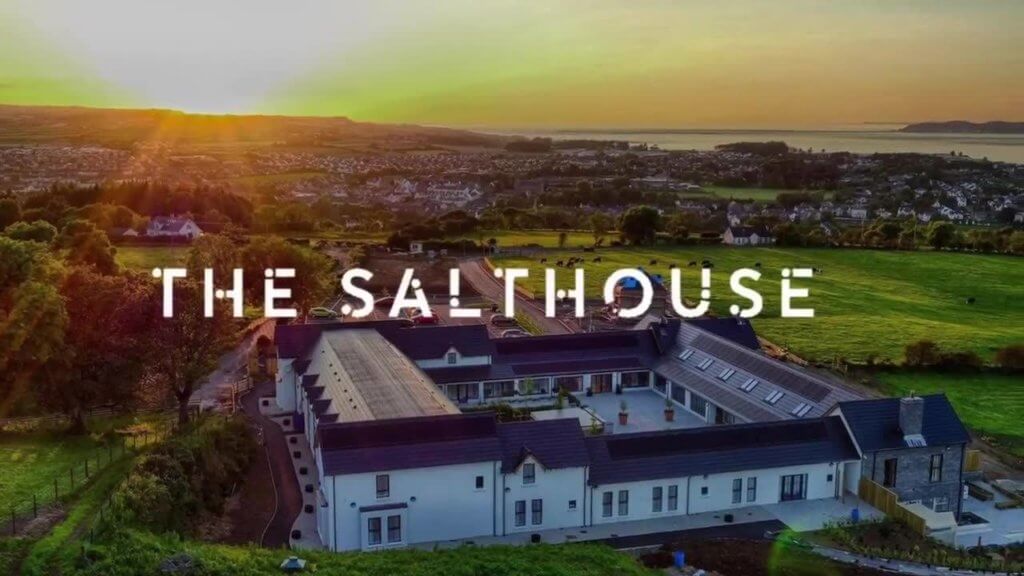This aerial photograph captures the large, square-shaped 'Salt House' building, characterized by a prominent inner courtyard. The building shows a mix of white walls and a gray roof, with the left and right wings appearing slightly larger. A notable feature is the gray section in the lower right corner, topped with a large stone chimney. The complex is surrounded by fields and scattered houses, while a body of water rests in the upper right corner, framed by rolling hills. The sky in the top third of the image is tinted with hues of chartreuse yellow and pale orange, suggesting a sunrise or sunset from the upper left. Sunlight streaks gently illuminate the scene. Overlaying the image is text in white capital letters reading "THE SALT HOUSE," adding a distinct touch to this tranquil landscape.